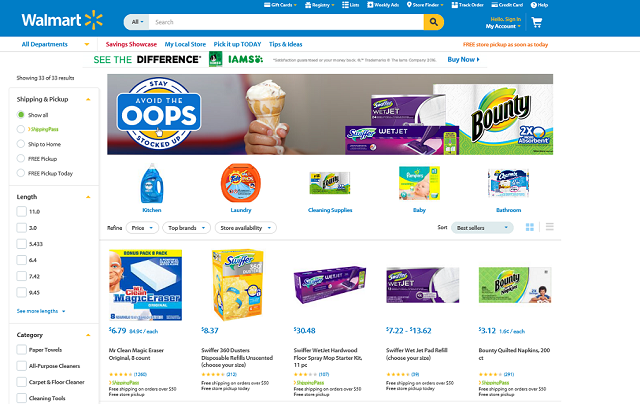The screenshot from a Walmart webpage captures the detailed layout and various sections of the online store interface. At the top of the screen, the Walmart logo is prominently displayed in the upper left corner, featuring white letters spelling out "Walmart" on a blue background, accompanied by a yellow sunburst with six rays. Adjacent to the logo is a search bar, followed by icons for "My Account," "Sign-In," and a shopping basket, all set against a continuous blue bar that spans the top of the page. 

Within this blue banner are additional tabs for "Gift Cards," "Credit Cards," "Track Order," and "Help." Below the blue bar, a secondary navigation bar includes tabs for "All Departments" with a dropdown, "Savings Showcase" highlighted in red, "My Local Store" in blue, "Pick It Up Today" also in blue, "Tips and Ideas" in blue, and on the far right, "Free Store Pickup As Soon As Today."

The main screen is highlighted by a banner at the top featuring the phrase "See the Difference" next to the IAMS logo, indicating a promotion for IAMS pet food, accompanied by a "Buy Now" button. Beneath this, a section on the left displays filtering options showing "11 of 13 results," with further selections for "Shipping and Pickup," including "Show All," "Ship to Home," "Free Pickup," and "Free Pickup Today." There’s also a selection of filter lengths listed as "11.0," "3.0," "5.433," "6.4," "3.42," and "9.45," with a "See More Lengths" option below. Categorization filters list "Paper Towels," "All-Purpose Cleaners," "Carpet and Floor Cleaner," and "Cleaning Tools."

The central portion of the screen is dominated by a banner image of a person holding a melting ice cream cone, with the text "Stay Stocked Up, Avoid the Oops" on the left, promoting a campaign for replenishing household essentials. On the right of the banner, images of household products like Bounty paper towels (advertised as "two times more absorbent"), Swiffer Wet Jet mop, and refills are displayed. Further down, various cleaning and household supplies are showcased, including categories such as "Kitchen," "Laundry," "Cleaning Supplies," "Baby," and "Bathroom."

Notable product listings include Mr. Clean Magic Eraser for $6.79, a Scuffer for $8.35, the Swiffer Wet Jet mop priced at $30.48, Swiffer Wet Jet refills ranging from $7.22 to $13.62, and a roll or package of paper towels for $3.12.